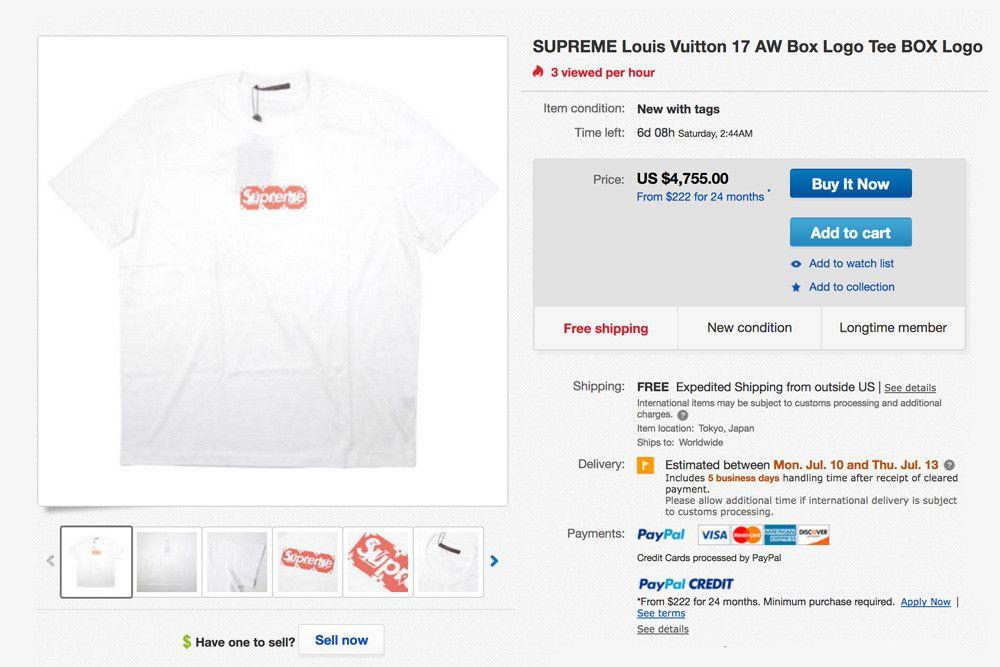This image captures an online product listing for a Supreme x Louis Vuitton 17 AW Box Logo T-shirt on a reseller platform like eBay. The page features a sleek gray background. Dominating the top left is a large square thumbnail showcasing the T-shirt neatly laid out flat. 

To the right of the image, the listing title reads "Supreme Louis Vuitton 17 AW Box Logo T-shirt" prominently. A red fire symbol next to the title indicates that the item is popular, stating "3 viewed per hour" in red text. Immediately below, the item condition is specified as "New with tags," with "New with tags" in bold for emphasis.

The listing highlights the remaining auction time as "6 days, 6 hours" with an end time of "Saturday, 2:44 p.m." Below this, a gray box details the pricing information. At the top left corner of the box, the price is listed as "U.S. $4,755." An optional financing plan is noted below, stating "From $222 for 24 months" in blue text.

To the far right within the gray box, large interactive buttons allow potential buyers to "Buy it now" (in dark blue) or "Add to cart" (in light blue). Below these options, smaller links offer the options to "Add to watch list" or "Add to collection" in small blue letters.

At the bottom of the gray box, additional product attributes are highlighted: "Free Shipping," "New Condition," and "Long-time Member"—with "Free Shipping" in red to catch attention.

In the bottom right corner of the listing, detailed shipping information is provided, outlining the delivery process and payment options. Accepted payment methods include logos for PayPal, Visa, PayPal Credit, MasterCard, American Express, and Discover.